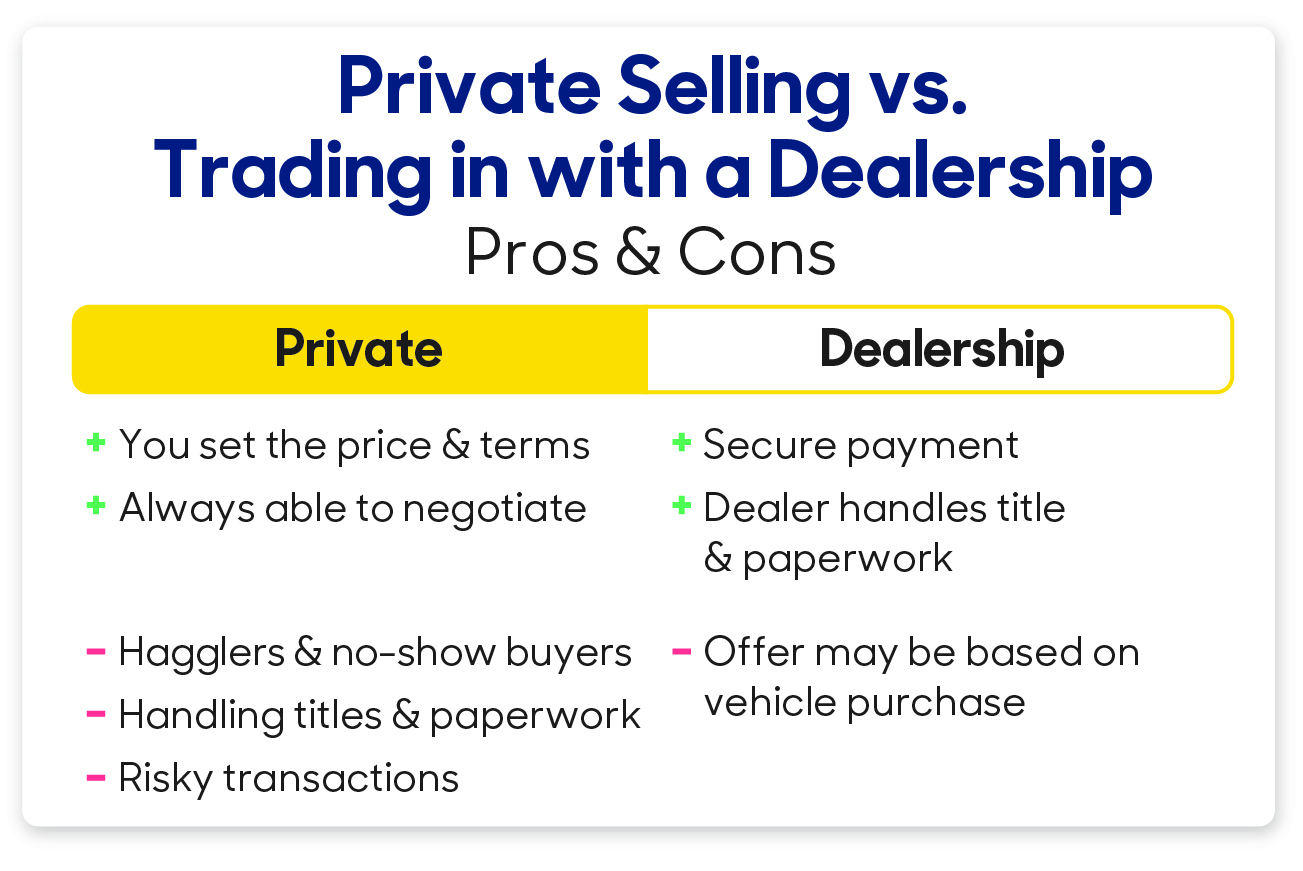The image is a computer screenshot, displaying a detailed comparison of private selling versus trading in with a dealership, highlighting the pros and cons of each. The title "Private Selling vs. Trading In with a Dealership: Pros and Cons" is prominently featured at the top in blue text. The background is white. 

On the left side, under the heading "Private," the pros include:
- Setting your own price and terms
- Constant ability to negotiate

These pros are bullet-pointed with green plus signs and highlighted in yellow. The cons, marked with red minus signs, include:
- Dealing with hagglers and no-show buyers
- Handling all titles and paperwork yourself
- Engagement in risky transactions

On the right side, labeled "Dealership" (also in a bluish color but not highlighted), the pros are:
- Secure payment
- Dealer manages title and paperwork

For the cons, the dealership has a single noted downside:
- Offer may be based on vehicle purchase

This clear and organized list uses contrasting text colors and bullet points to emphasize the different factors to consider when choosing between private selling and trading in with a dealership.